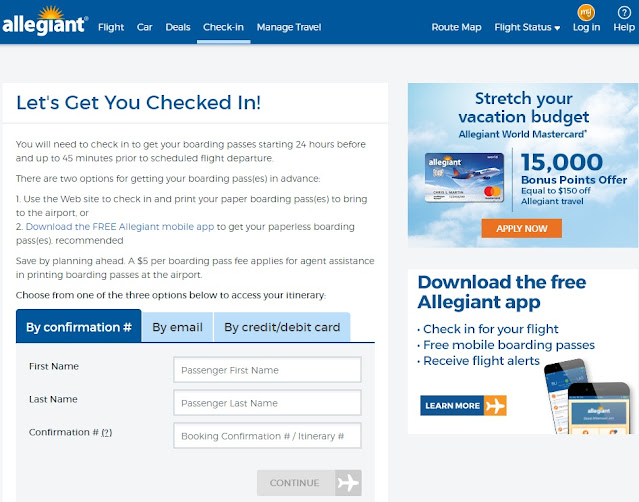The image depicts a travel planning website with a user interface geared towards facilitating flight check-ins. Dominating the top of the page is a prominent blue border, housing essential information in white lettering. The brand "Allegiant" is displayed in bold, small letters with a distinctive yellow sun icon emerging from the "G" in "GIANT." 

Adjacent to the brand name, a series of navigational tabs are sequentially aligned: "FLIGHT," "CAR," "DEALS," "CHECK IN," and "MANAGE TRAVEL." Notably, the "CHECK IN" tab is underlined with a light-colored line, indicating the current selection. Over at the far right of the blue border, additional options appear: "ROUTE MAP," "FLIGHT STATUS" with a dropdown arrow icon, "LOGIN" with a yellow circle icon, and "HELP" signaled by a blue circle encompassing a white question mark.

The main content area is headed with the message, "Let's get you checked in," followed by instructions noting that passengers must check in to obtain their boarding passes from 24 hours before and up to 45 minutes before the scheduled flight departure. Further details on the check-in process are provided below this message. 

At the bottom of the screen, there is a text entry confirmation box prompting users to input their first name, last name, and confirmation number. It also offers alternative methods for locating the boarding pass; users can choose to search by confirmation number, by email, or by credit/debit card.